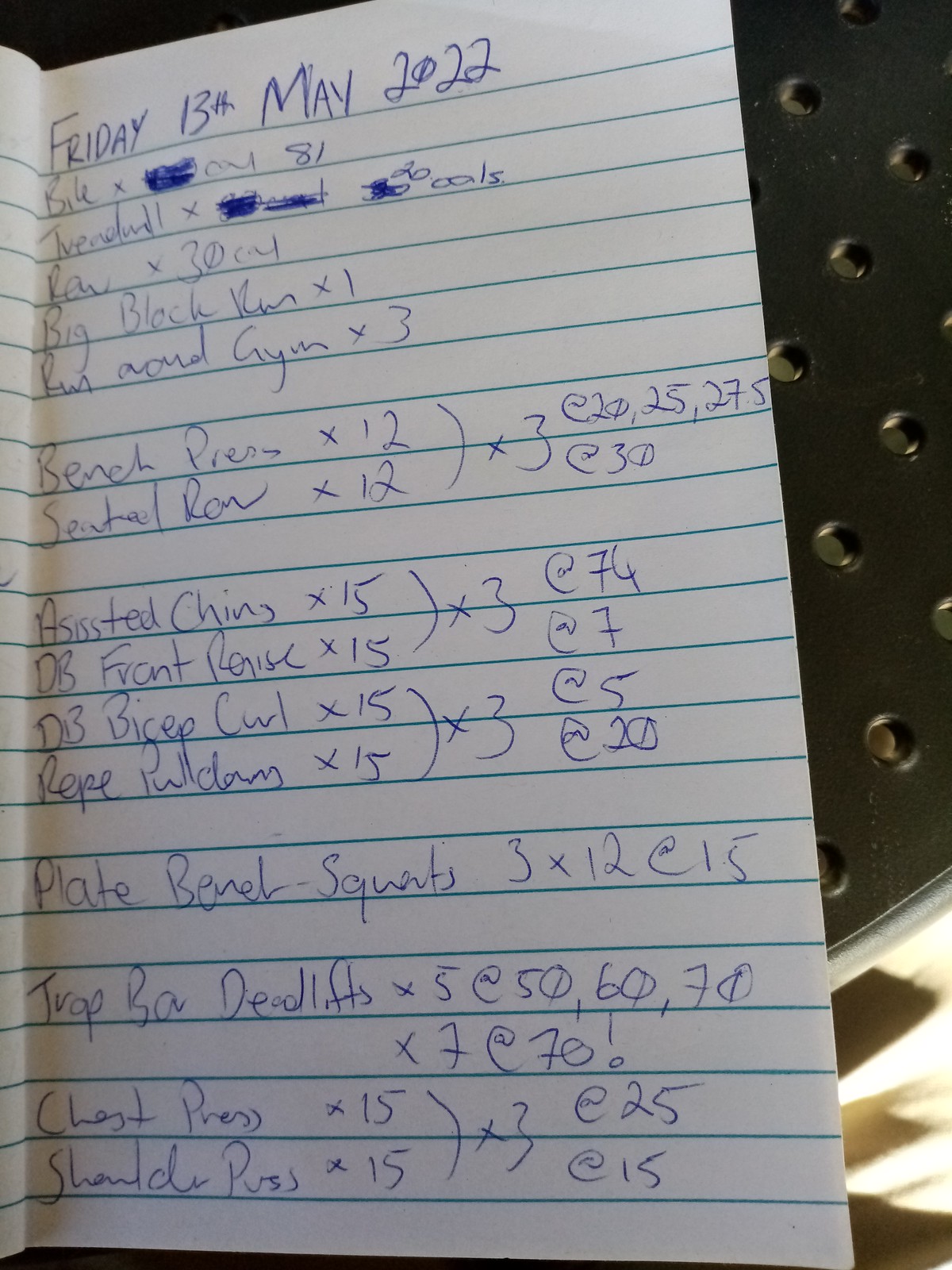The image depicts a detailed workout plan handwritten in blue ink on white paper with green lines. Dated at the top as "Friday 13th May 2022," the plan outlines various exercises and their repetitions. The first line lists "bio times cal 81" followed by sequences such as "10 mil times 20 cals" and "more times 30 cal." It includes specific exercises like "big rock rm times one," "run around gym times three," and "bench press times 12," followed by "sit down row times 12" grouped in a bracket indicating this should be repeated three times. The list continues with "shoulder press times 15" at the bottom. Notably, the paper is placed on a black metal surface with perforated dots. The detailed notes appear to be part of a structured training regimen, possibly for a fitness enthusiast or trainer.